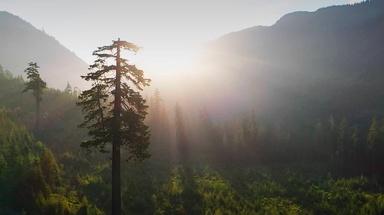In this captivating photograph taken in nature, the bright Sun is positioned between two mountainous areas, either rising or setting, casting a dramatic light across the landscape. The sunlight is piercing through the mist and creating striking "God rays" that streak downwards. The sky above the mountains is a muted grayish-blue, contributing to a beautiful contrast in the image. The mid-ground features a lush green expanse with some yellowing foliage, composed of grass, treetops, and shrubs. Dominating the scene near the center is a particularly tall tree with sparse branches, possibly a pine or evergreen, standing out against the background of other trees. The vibrant greenery of the valley adds to the enchanting view, making the whole scene appear both serene and awe-inspiring.